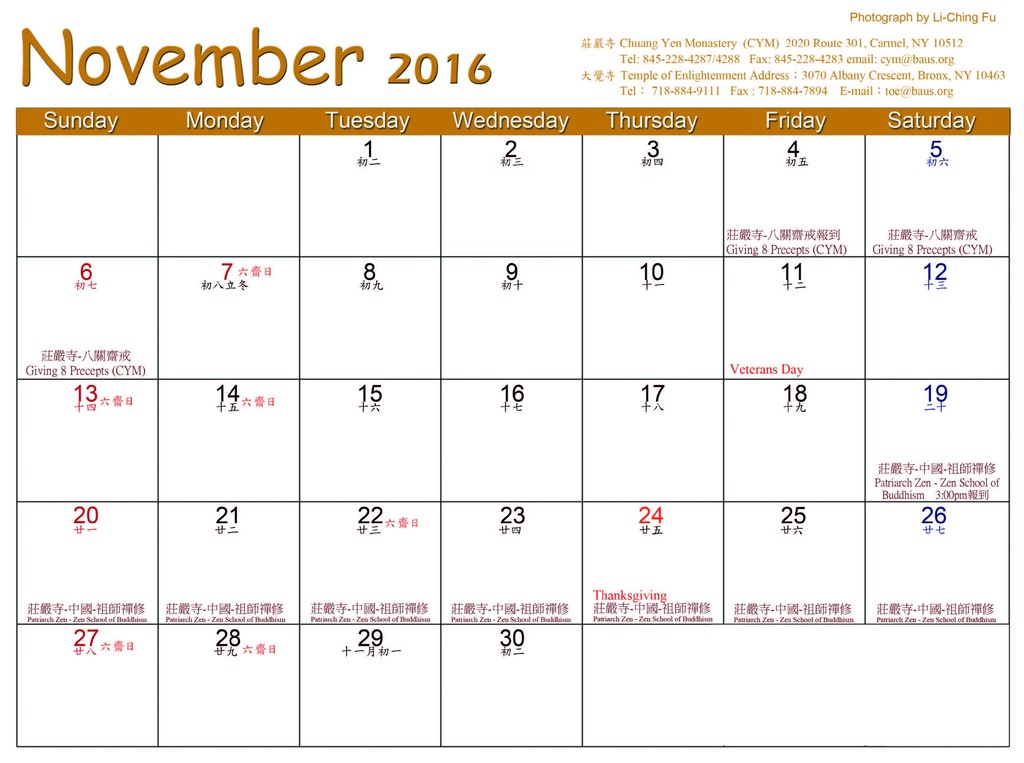This image features a calendar for November 2016. The calendar starts with the 1st on a Tuesday and runs through to the 30th. The overall background is white, with dates primarily in black, while some dates are highlighted in red and blue. Across the top left, the text "November 2016" is displayed in a goldish-autumn tint, which matches the days of the week that are listed from Sunday to Saturday in a gold bar at the top. The top right corner bears the text "Photographed by Li Ching-Fu," along with additional information such as "Chengyin Monastery, CYM 2020, Route 301, Carmel, New York, 10512."

The dates on the calendar include both English and Chinese characters, with Chinese writing beneath each date, likely specifying the day's number. Noteworthy entries include Veterans Day on the 11th, marked clearly in red, and Thanksgiving on the 24th. Additionally, there are annotations in blue on dates like the 4th, 5th, and 6th, which note the "giving 8 precepts" with the abbreviation "CYM." The detailed layout and bilingual elements provide a rich, cultural touch to the calendar's design.